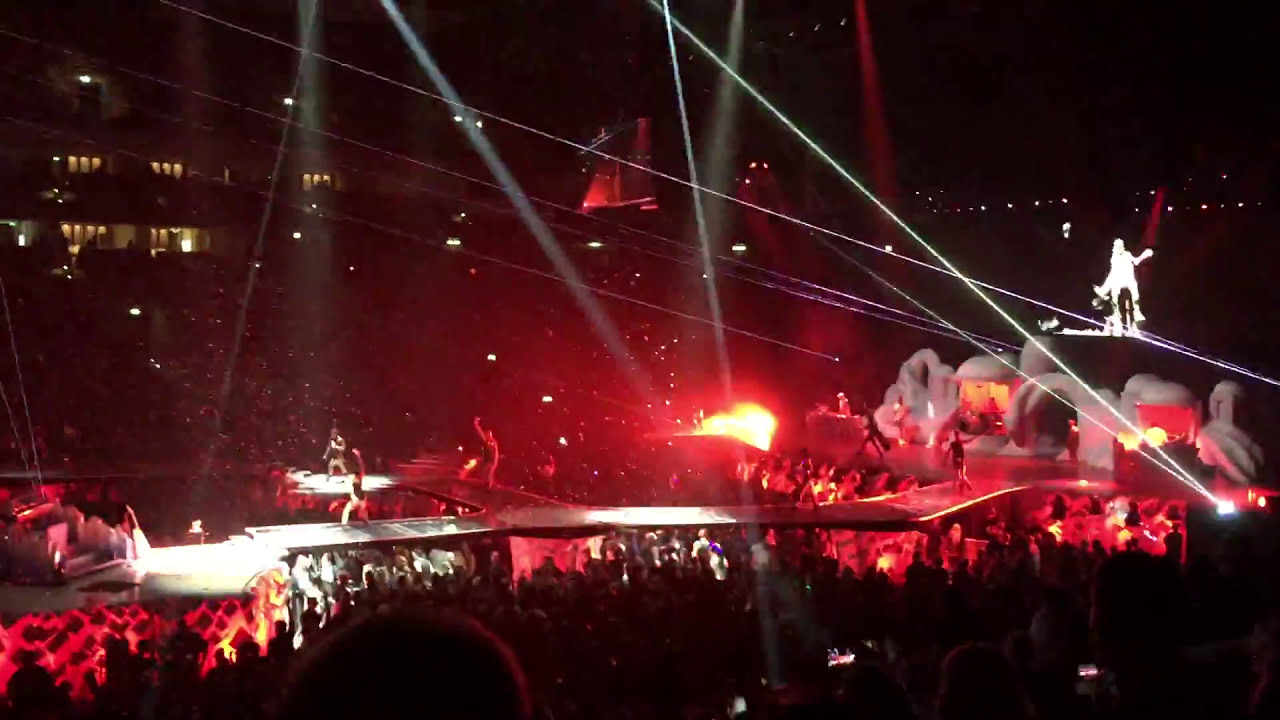The image depicts a dynamic outdoor concert set against the backdrop of apartment buildings. The stage, positioned in the bottom third of the image, extends from left to right and features performers engaged in a lively act illuminated by vibrant lighting. A dark crowd fills the area below and above the stage, blending into the shadowy background. The scene is accentuated by dramatic spotlights creating streaks of red, white, and black light across the image. The back of the stage is decorated with white, large, domed set design props, giving a cartoon-like, almost surreal quality to the setting. To the right of the stage, there are curved, elevated structures that seem to serve as walkways or additional viewing areas, with a performer highlighted under the spotlights. The overall atmosphere is one of an energetic nighttime event with an array of lights and shadows contributing to its vivid, almost ethereal visual impact.